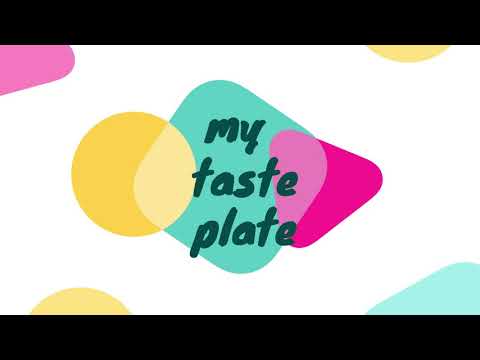The image features a simplistic yet vibrant design with a black header and footer framing a white background. In the upper left-hand corner, there is an elongated pink bubble-like spot. The upper right-hand corner shows half of a yellow circle, while the lower left-hand corner has a similar light yellow half circle. In the lower right-hand corner, a light blue oblong spot can be seen.

At the center of the image lies a composition of shapes overlaid upon each other: a yellow circle is superimposed over a blue diamond with rounded corners, which in turn overlays a pink triangle also with rounded edges. Central to the design is the text "my taste plate," written in lower-case dark blue lettering, arranged vertically with "my" above "taste," which is above "plate." 

The overall arrangement and choice of colors—yellow, pink, and blue with their respective shades—give the impression of minimalist digital art, possibly serving as an introductory slide for a video.